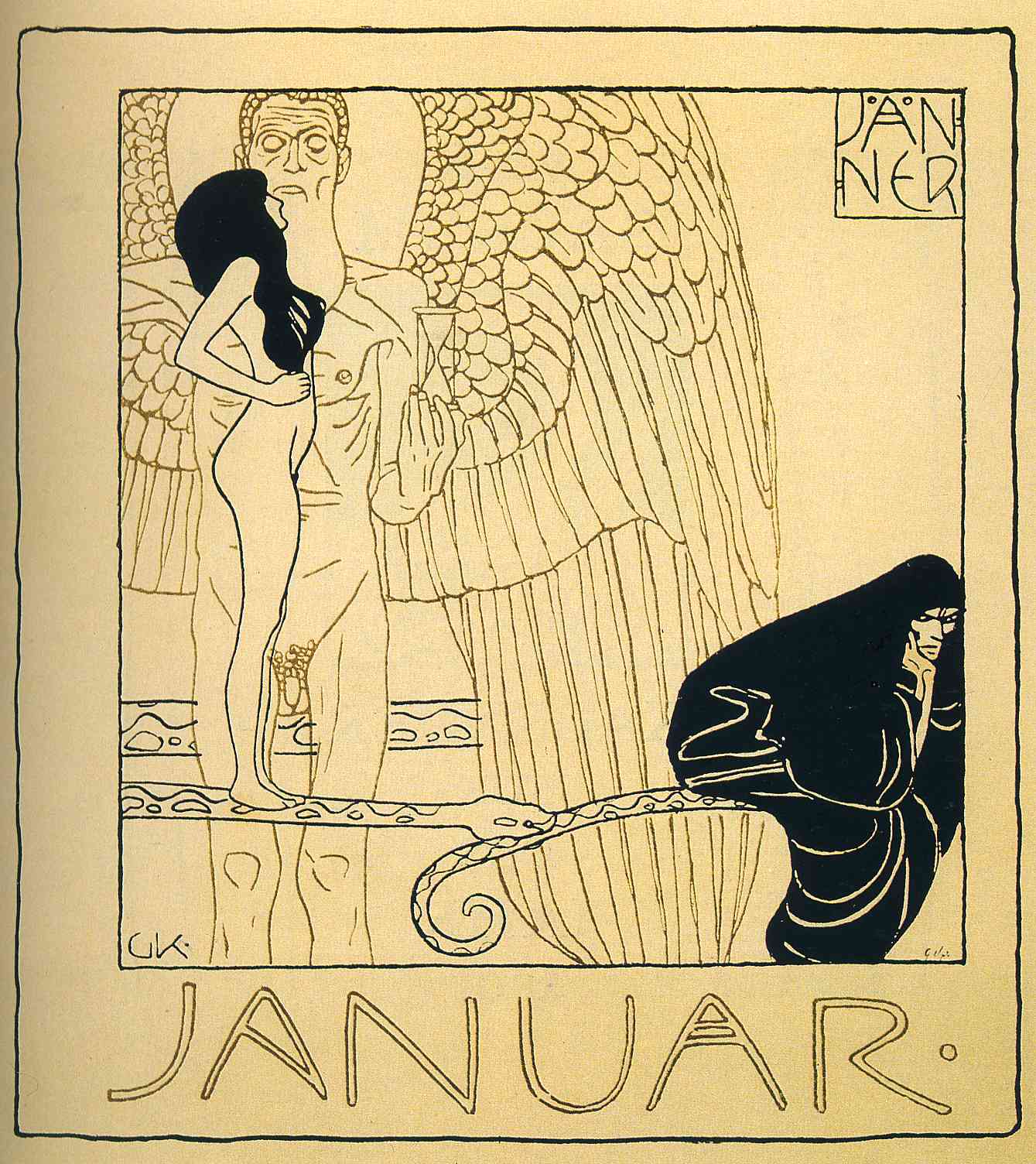This aged, cream-colored line drawing, created in a light brown and blue ink, portrays a mythological scene. At the center, a nude male figure with expansive angel wings stands prominently, holding an hourglass. Enveloped by a coiling snake, which bites its own tail, this angelic figure faces forward, his wings dominating the composition. To his left, a nude woman with long, dark hair, sufficient to modestly cover her breasts, stands on the snake’s back, looking upward in profile. On the snake’s lower right side, a dark hooded figure sits, draped ominously in black, conveying a sense of displeasure or malevolence. The word "Januar" is inscribed in both the lower right and upper right corners of the piece, suggesting a date or title in another language, likely Latin, enhancing the enigmatic and mythic quality of the illustration.